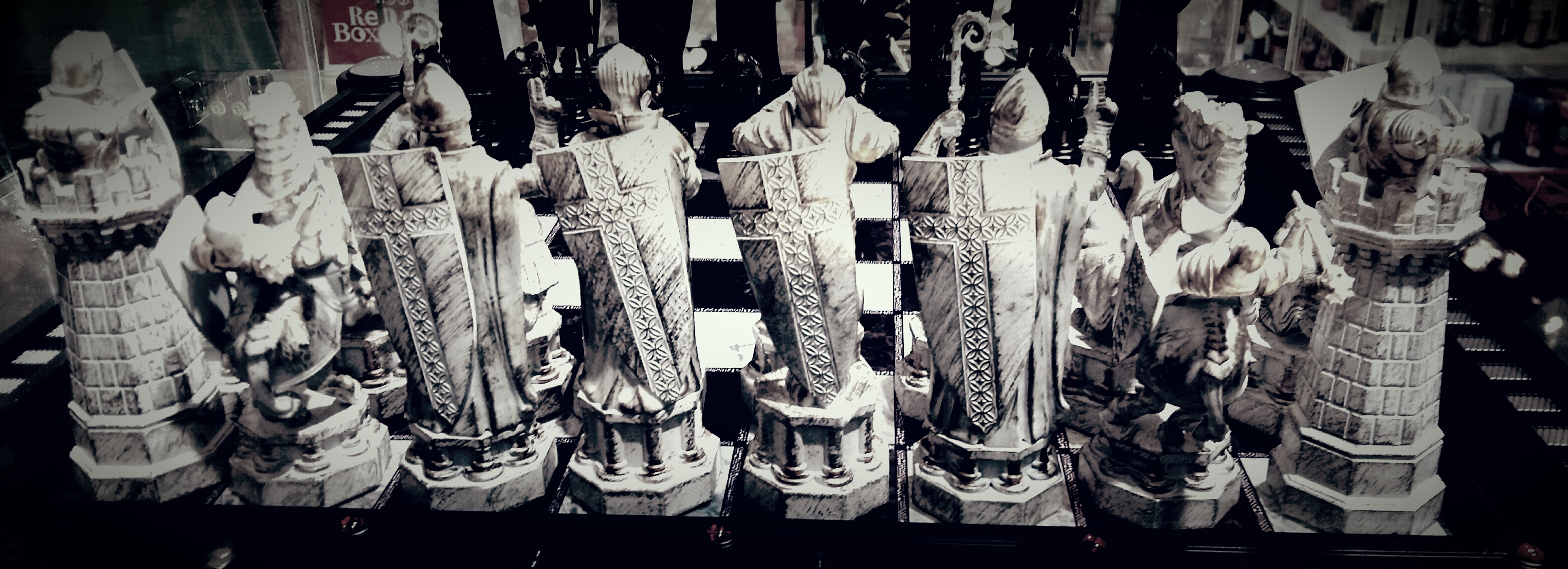This is a black-and-white close-up photograph of a highly ornate and stylized chess set, focusing on the white pieces at the front edge of the chessboard. The photograph highlights the exquisite detail of each piece, with the rooks resembling castles, and the bishops, king, and queen featuring shields on their backs. Some of the pieces also appear to be holding weapons in their right hands. The knights are intricately designed and hard to discern due to their complexity. The chessboard, which spans eight squares across, has its black pieces faintly visible in the background. The lighting in the photograph is strongest in the middle, gradually dimming toward the edges, making it difficult to identify the surrounding environment. There is a hint of red in the background, adding a subtle accent to the overall monochromatic image. The scale of the chess set is indeterminate from the photograph alone.